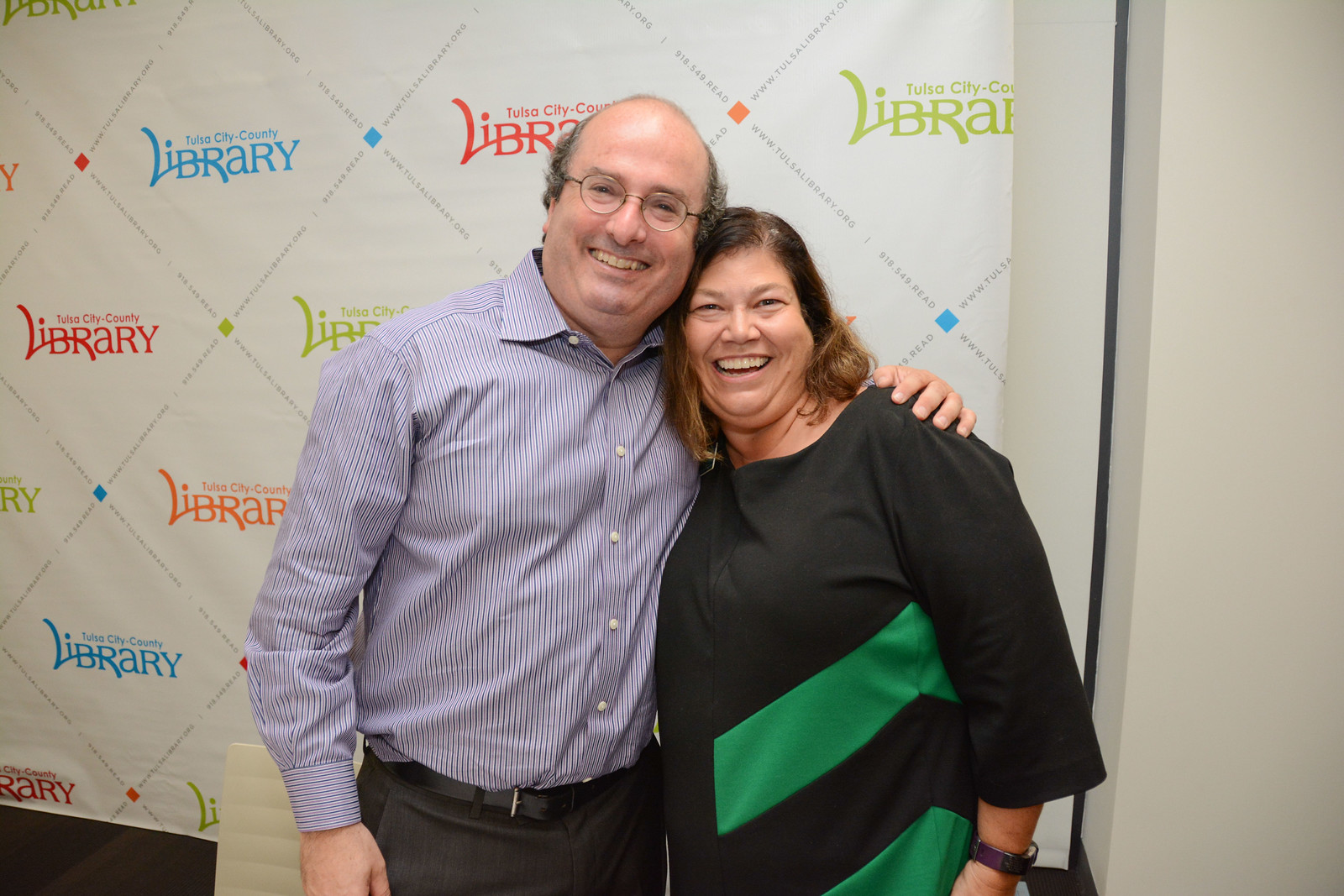In this color photograph, a middle-aged man and woman are standing closely together, smiling at the camera with a cheery demeanor. The man, positioned on the left, is gently balding with some gray hair, and he is wearing round glasses. His attire includes a purple pinstriped, collared dress shirt with white buttons that is slightly open at the neck, and slate gray dress slacks held up by a black belt. He is also wearing black shoes. With a warm smile showing his teeth, he has his arm affectionately wrapped around the woman beside him. 

The woman, who sports medium brown hair parted to the side, is beaming widely with her teeth visible. She is dressed in a mostly black top that features green accent stripes along the sides. A watch adorns her wrist. Both of them radiate happiness and comfort with each other, as they pose in front of a bright, multicolored backdrop. This backdrop prominently displays the text "Tulsa City County Library" in a mix of blue and green, followed by red and orange, with the words set against a simple white background. Behind them, the white walls of the room are visible, suggesting they are likely inside the library where the display is set up.